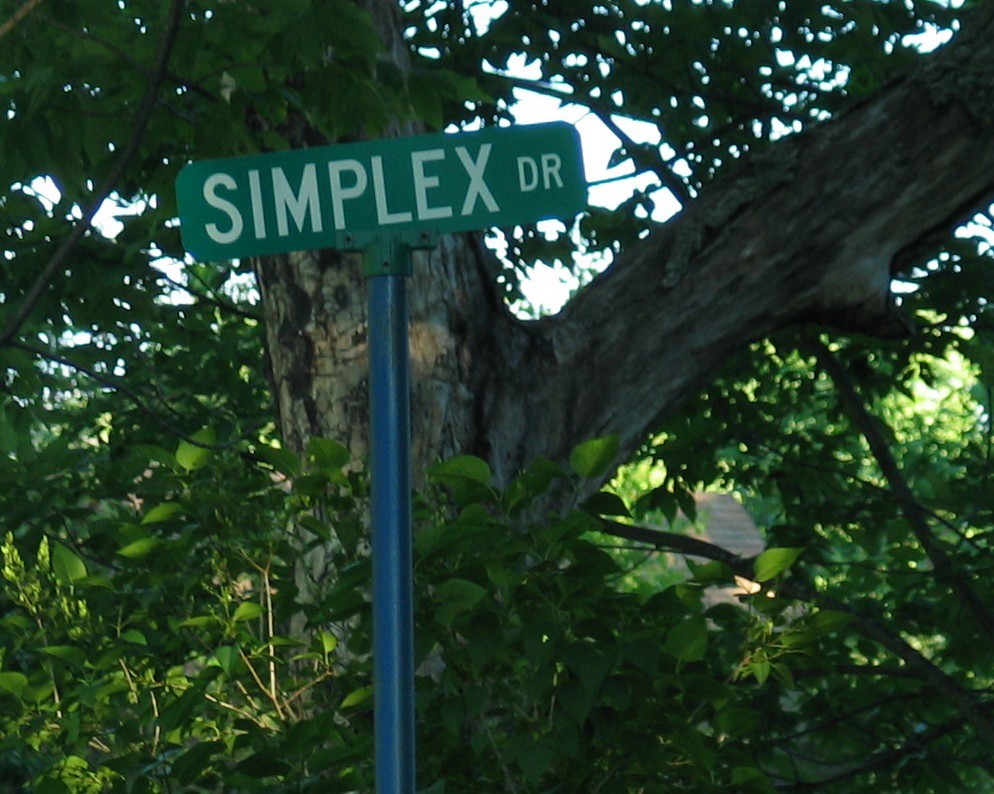The image features a metal pole painted blue, supporting a small, green street sign with crisp, white lettering that reads "Simplex Dr." The sign is affixed horizontally, indicating the name of the street. Behind the sign stands a majestic, mature tree with a textured bark exhibiting shades of brown, gray, lighter hues, and even some reddish tones. The tree's foliage is abundant and vibrant, with small, healthy leaves in a deep green color, creating a lush canopy. Beneath the tree, a rippling gray body of water is faintly visible, suggesting a serene setting. The sky overhead is overcast, casting a soft, grayish glow across the scene, adding to the tranquil atmosphere.